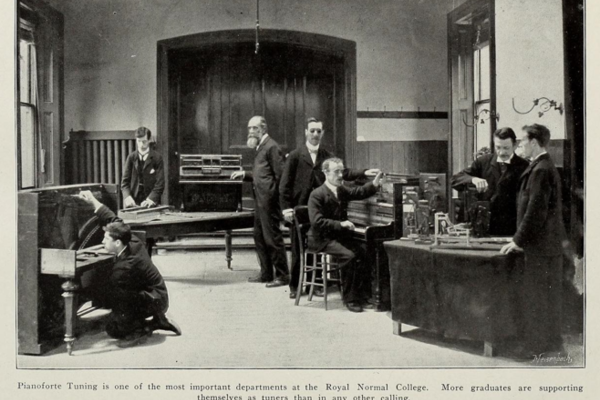This antique black-and-white photograph, likely a dated image from a newspaper clipping, captures a significant moment at the Royal Normal College, specifically within the renowned Piano Forte Tuning department. The image features seven men, all dressed in dark suits with white collars, some with beards and mustaches. On the left, a man is crouched down, intently peering into a piano, possibly tuning it. Behind him, another piano-like system is attended by two men; one, bald with a bushy beard, and the other, with brown hair, are standing next to a radiator. To the right, four men are gathered around a large table cluttered with unidentifiable equipment. The room is minimally decorated, focusing primarily on the furniture and equipment essential for their work. The caption at the bottom reads: "Piano Forte Tuning is one of the most important departments at the Royal Normal College. More graduates are supporting themselves as tuners than in any other calling." Sunlight filters through windows on either side of the room, illuminating the diligent efforts of these men in their craft.